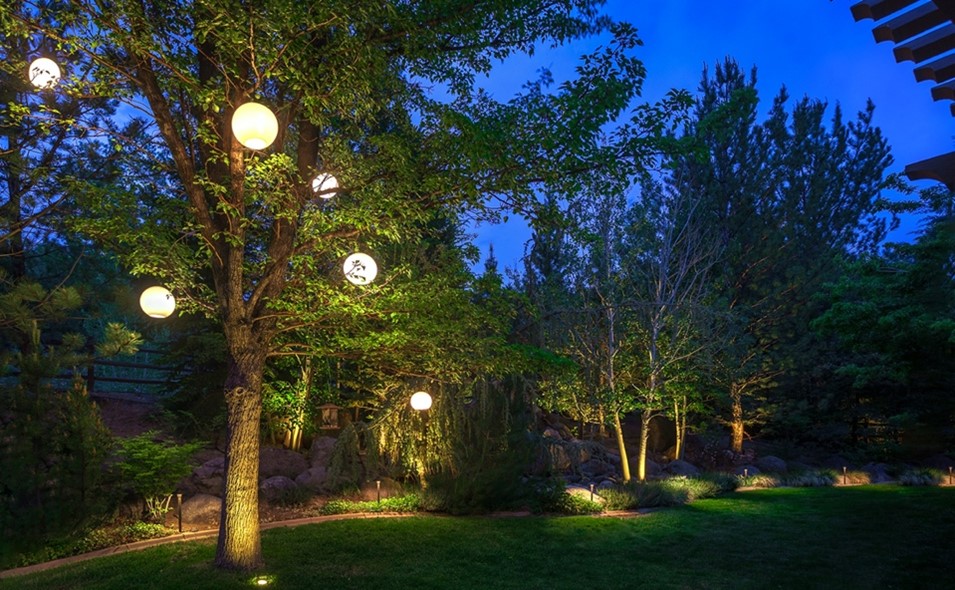The image captures a beautifully maintained garden space, photographed shortly after sunset during twilight. The meticulously manicured lawn is bordered by a small brick perimeter, beyond which lie short hedges and clumps of grass. Dominating the scene is a tall tree adorned with glowing Japanese paper lanterns, casting a warm yellow light. Additional solar stake lights illuminate the perimeter of the lawn. The sky in the background is a rich, dark blue, adding to the tranquil ambiance. Behind the grassy area, there is a subtle slope leading up to a wooden fence. The overall scene is serene and well-lit, emphasizing the care taken in maintaining the garden’s aesthetic.